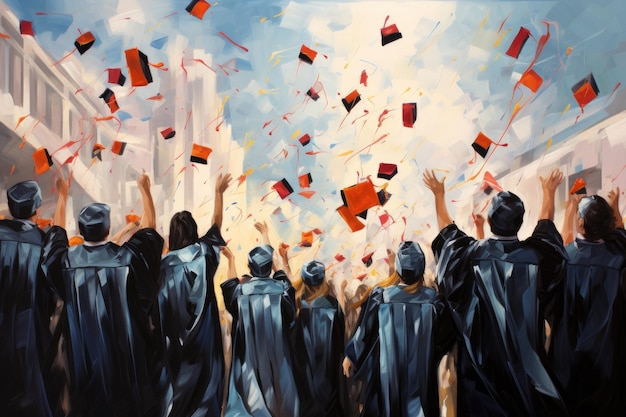The image is a detailed and vibrant depiction of a graduation celebration, likely rendered in watercolor or pen and ink. The illustration presents about nine graduates, seen from the back, joyously throwing their red and orange mortarboards into the air against a backdrop of a bright, partially cloudy blue sky. The graduates are dressed in dark blue or black gowns, with most of them also wearing another type of blue hat underneath their mortarboards, suggesting possibly doctoral attire. Their arms are jubilantly raised, capturing the moment of celebration and accomplishment. The background features abstractly painted smudged white buildings on either side, emphasizing that the focus is on the animated and lively celebration of the graduates. Confetti seems to drift through the air, adding to the festive and exuberant atmosphere of the scene.